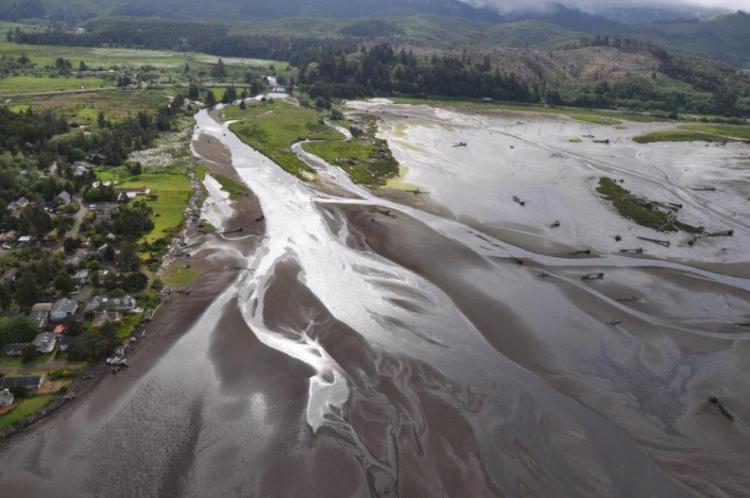The aerial photograph captures an expansive river delta, likely taken from a drone or a plane, showcasing an impressive view from high above. In the background, foothills of lush, green mountains rise up, capped with low-lying clouds. The delta spans from the top left corner to almost the entire bottom right, where the river, characterized by its muddy brown waters, discharges into a wide basin, creating intricate rivulets that cut through the muddy flats.

In the upper left, the muddy water is interspersed with black objects and a small, green island-like space. Along the left-hand side of the image, a small town can be seen nestled in a heavily forested area. The town is dotted with houses bordering the water and has a central street threading through the community. On the right side, the muddy waters intrude towards the green parts of the town, where more pristine buildings are scattered amidst the trees. A clearly visible road heads towards the upper right, further emphasizing the blend of natural and urban landscapes in this richly detailed scene.